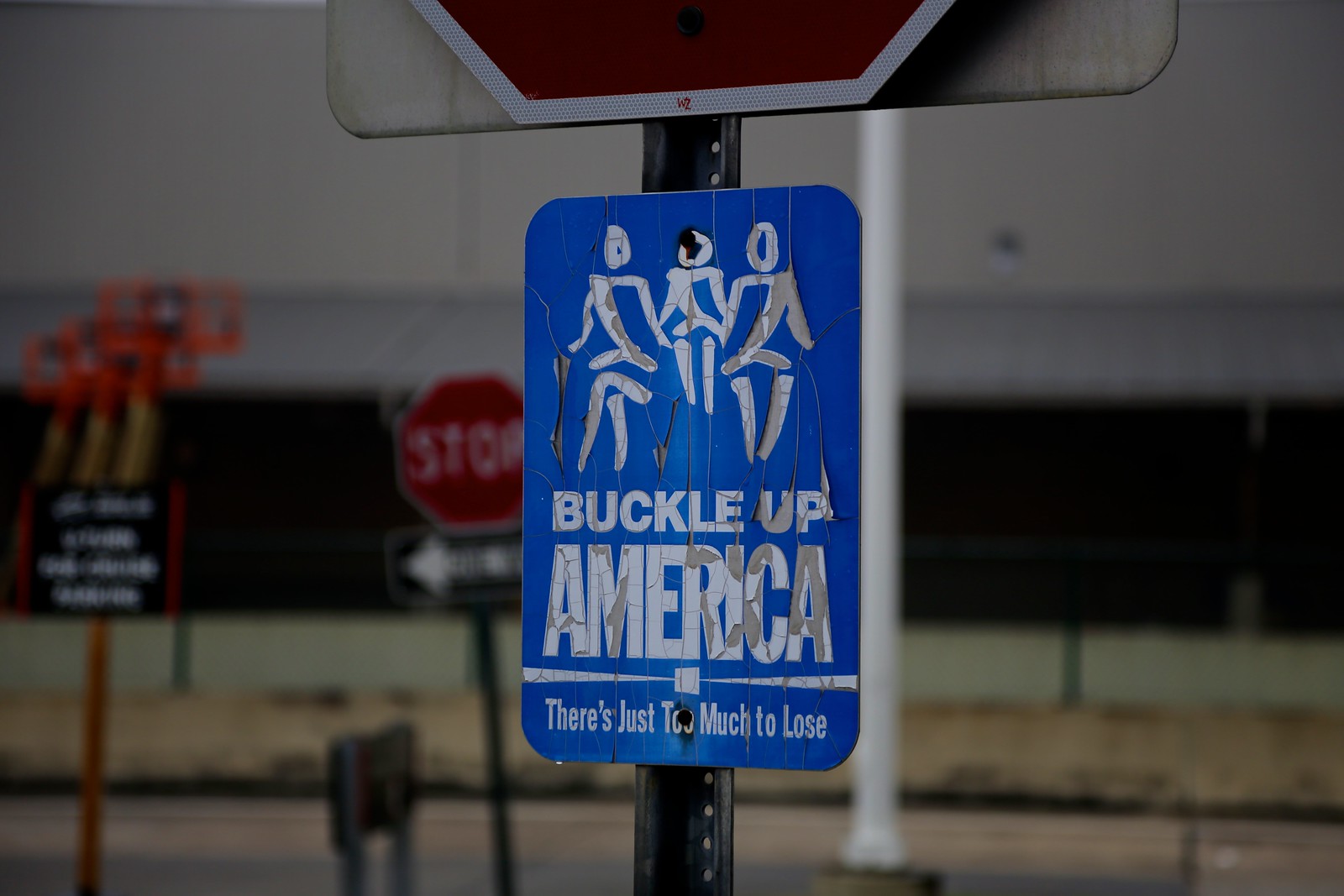This detailed close-up photograph captures a blue sign with white text and illustrations, positioned on a pole directly beneath a stop sign. The blue sign prominently displays the message "Buckle Up, America. There's just too much to lose," accompanied by a caricature of three stick-figure people—two adults seated in the front and a child in the back—all wearing seat belts. The surrounding environment is slightly out of focus but suggests an urban setting, with additional road signs visible, including another stop sign and a one-way sign pointing to the left. The blurred background hints at a road and possibly the side of a building or a bridge-like structure. The emphasis on safety and seatbelt use is clear amidst the various street signs dispersed in this roadside scene.